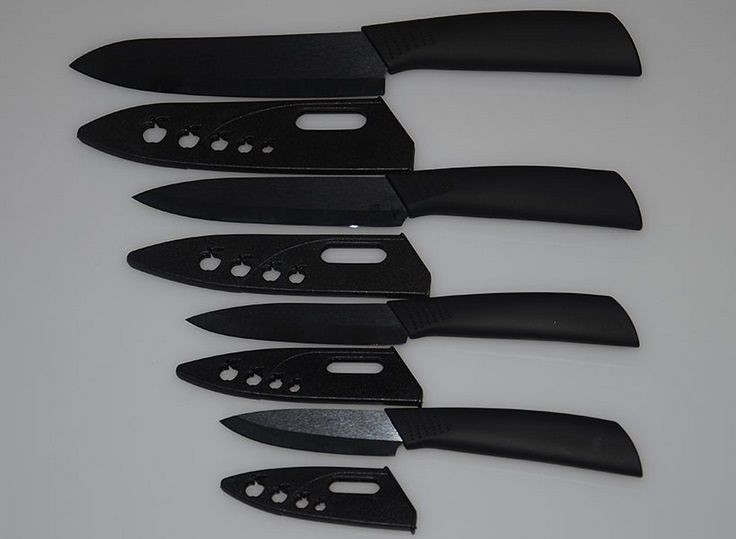The image displays a set of four different-sized cooking knives laid out on a white background. Each knife features a black rubber handle and a sharp, black-colored blade. Beneath each blade, there is a corresponding plastic sheath designed to protect the blade and the user. These sheaths have hollowed-out sections, allowing visibility of the blades while ensuring safety. The largest knife, placed at the top, has a sheath with five apple-shaped holes, while the sheaths for the three smaller knives each have four apple-shaped holes. The knives are arranged in ascending order of size from the bottom up, starting with the smallest, likely a paring knife, and going up to the largest. The design suggests that the knives may be customizable or interchangeable, although each knife appears fixed in the image.